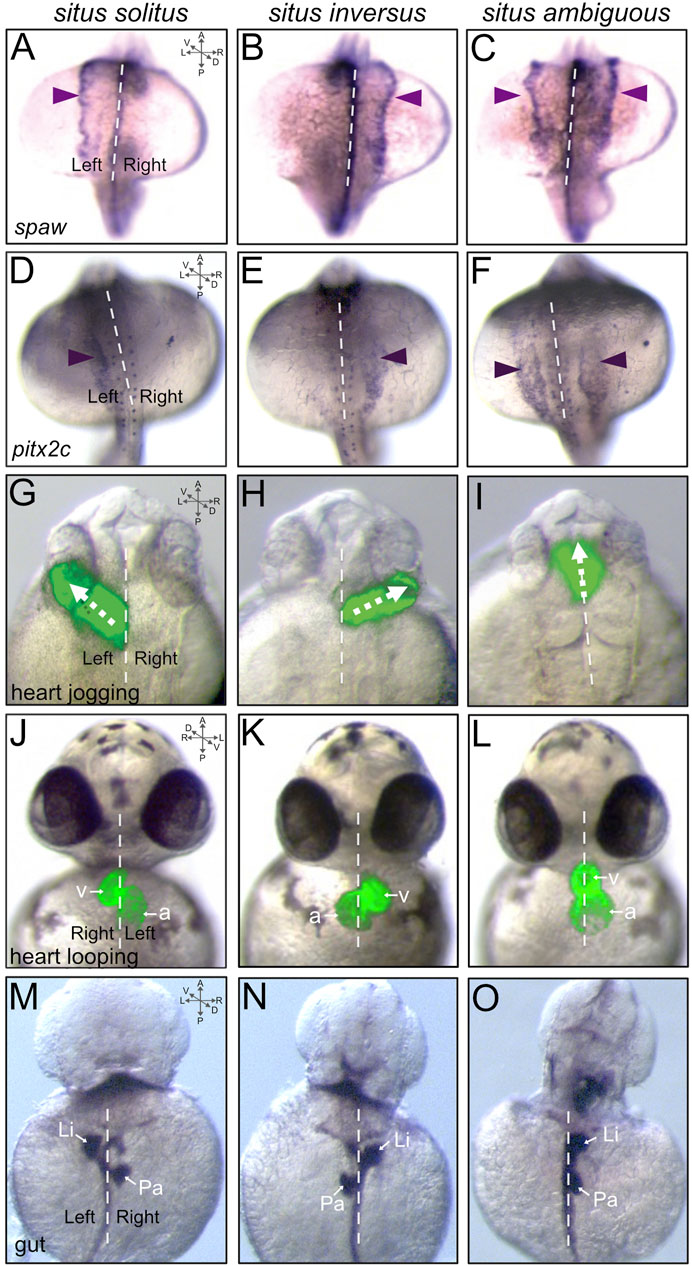The image displays a detailed scientific diagram titled "Cetus Solitis," "Cetus Inversus," and "Cetus Ambiguous" at the top. This diagram is organized into five rows and three columns, each column labeled with one of the aforementioned titles. Each row contains different types of illustrated creatures that appear to range from marine animals to insects, such as fish, jellyfish, birds, and bugs with distinctive big black eyes and white bodies. Notable labels, including "spa," "pix2c," "heart jogging," "heart looping," and "gut," are distributed across the rows and columns, indicating various observation points or stages. Each row's images depict left and right views of these organisms. The diagram intricately displays over 15 different creatures, with each column representing a variation in their physical structure or orientation, all meticulously laid out in labeled panels to emphasize the diversity and complexity of these specimens.